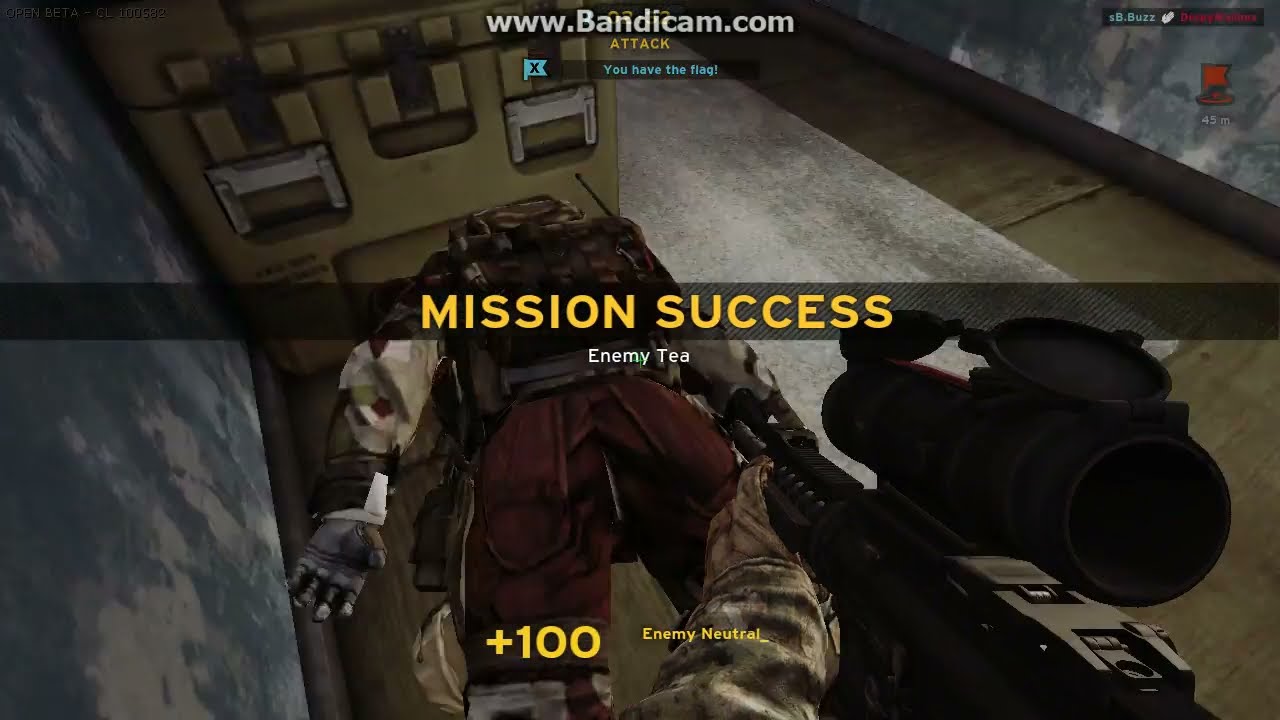This screenshot, captured from a gameplay video on www.bandicam.com, showcases a first-person shooter video game in the midst of a multiplayer match. The scene is set in a dimly lit room with some light patches highlighting the dark brown floor. The game's interface displays that the players are on round 8 of 15. In the top right corner, bold gold lettering indicates the current objective: "DEFEND," where players must prevent the enemy from extracting the flag. Beneath this objective, team scores are shown with Bravo Team 6 in light blue and Alpha Team 1 in red. On the left side of the screen, there's a Loadout section detailing the player's equipment, including a primary assault rifle with a mounted scope, an M9 pistol as the secondary weapon, and two types of grenades—a standard grenade and a stun grenade. The comprehensive loadout suggests that players can choose among a wide variety of weapons and accessories, emphasizing the customizable nature of the game.